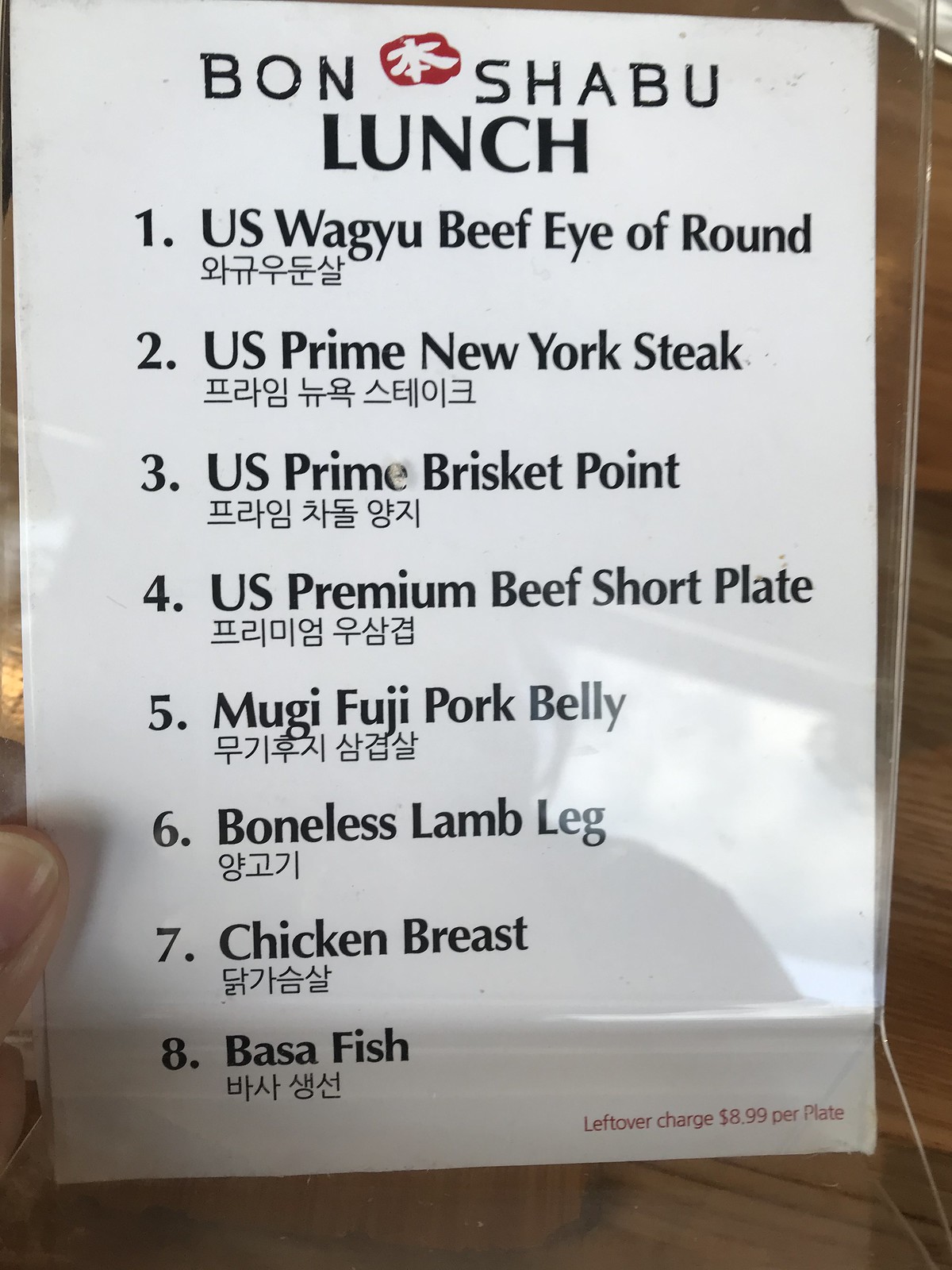In this image, a person is reading a menu that appears to be displayed on a clear glass door. The menu is white with black text, and it seems to belong to a Japanese steakhouse named "Bon Shabu Lunch." The language used for item descriptions and prices is not understood by the reader, but there is a clear numbered list from one to eight. The items listed are:

1. U.S. Wagyu Beef Eye of Round
2. U.S. Prime New York Steak
3. U.S. Prime Brisket Point
4. U.S. Premium Beef Short Plate
5. Mugi Fuji Pork Belly
6. Boneless Lamb Leg
7. Chicken Breast
8. Basa Fish

Each item is accompanied by text in what appears to be Japanese, possibly indicating the price for each dish. Between the words "Bon Shabu," there is a logo in Japanese writing. Additionally, at the bottom right-hand corner of the menu, there is a notice stating a "leftover charge" of $8.99 per plate.